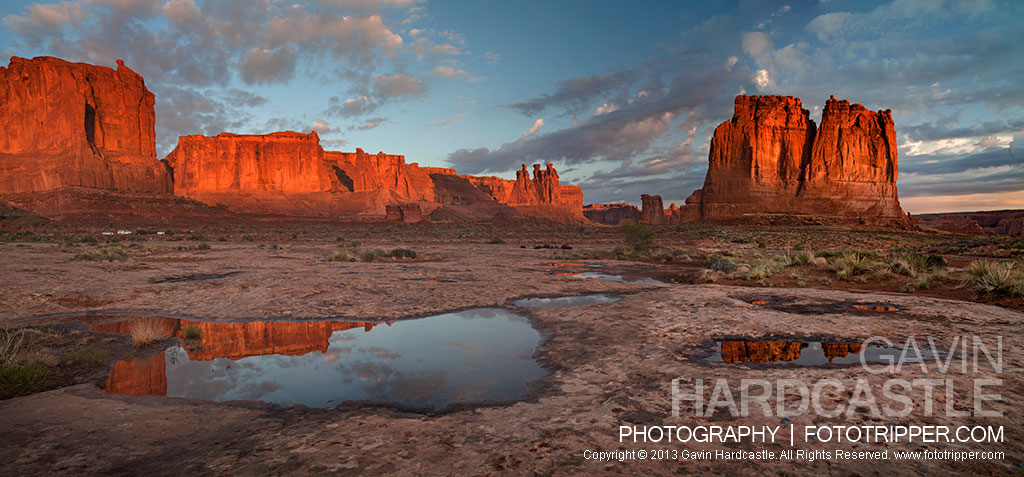This panoramic photograph captures a stunning desert landscape, likely taken during sunset. In the foreground, patches of dry dirt and scattered cacti give way to shallow puddles of water, which reflect the orange-tinged clouds and rock formations, adding a surreal beauty to the scene. The midground features low-growing, shrub-like vegetation leading up to an array of striking rock sculptures—two taller structures on the left and right sides framing a wider, flatter one in the center. The sky above is a mix of soft blue and gray clouds, tinged with warm hues from the setting sun. The bottom right corner of the photo bears the watermark and credit: "Gavin Hardcastle Photography, phototripper.com, copyright 2013 Gavin Hardcastle, all rights reserved, www.phototripper.com." This detailed and atmospheric image epitomizes the stark and captivating beauty of the desert.